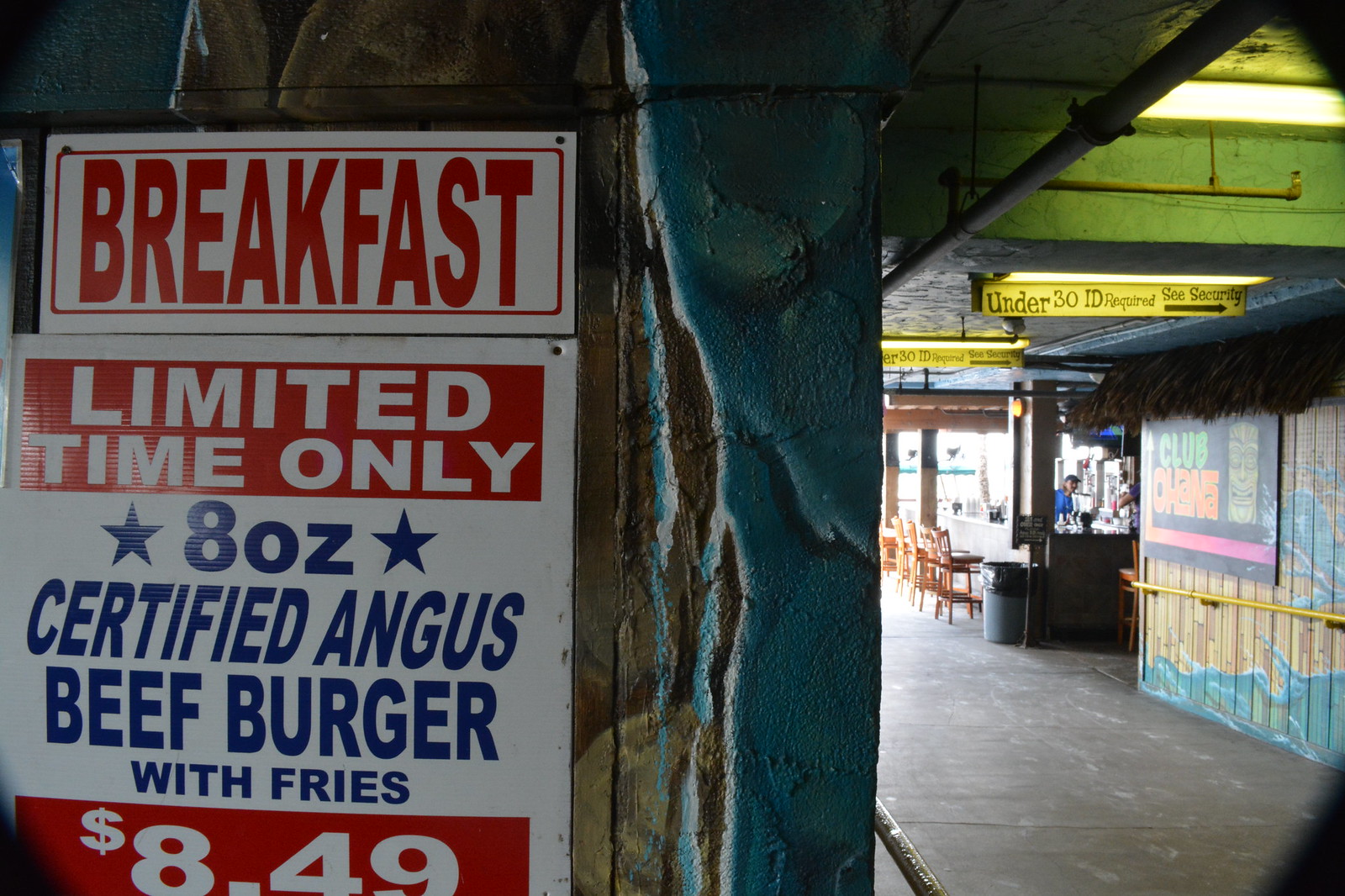This image captures the interior of a restaurant, showcasing a blend of its diner and bar areas. On the left-hand side, a prominent sign on the wall catches the eye, titled "Breakfast" in white letters on a red background. Beneath it, the sign advertises a limited-time offer for an 8-ounce certified Angus beef burger with fries, priced at $8.49, presented in a red box. To the right, an opening leads to another section of the restaurant where a bar with wooden stools is visible. Behind the bar, a person in a blue shirt and matching cap stands, suggesting a typical workday setting. Adjacent to the bar on the right, there's a painted wall featuring a handrail and partially visible signage starting with "Club". Hanging from the ceiling, a sign mandates "Under 30 ID required", hinting at the establishment's age policy. Sunlight streams through the windows at the back, indicating a bright day outside, further illuminating the scene. The atmosphere implies a typically busy space now captured in a moment of stillness, with no patrons currently in view.